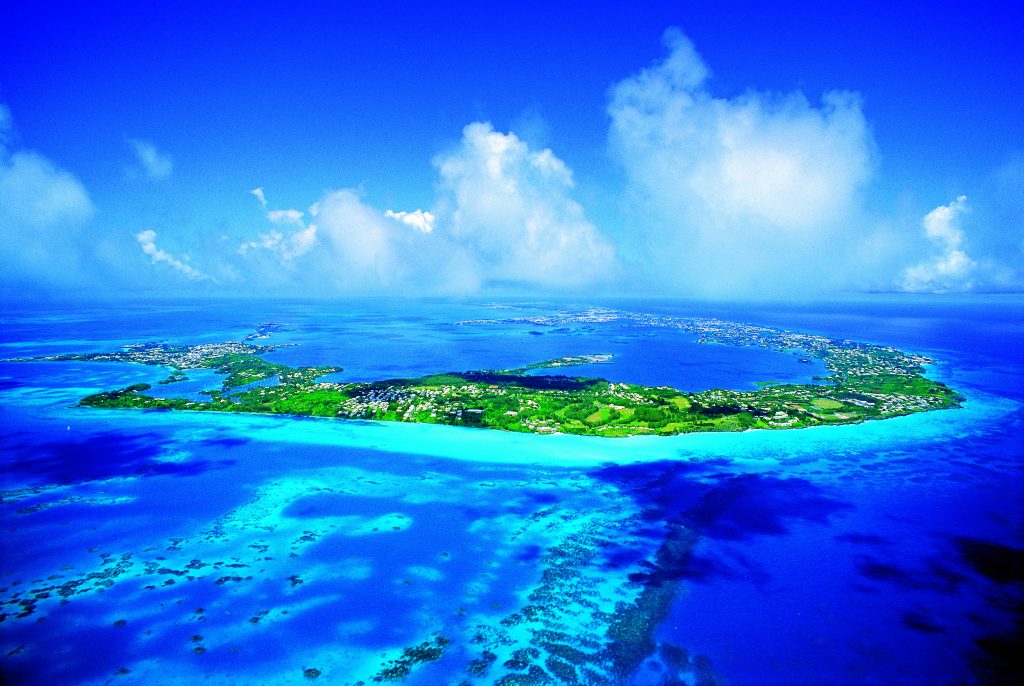This photograph captures a striking aerial view of a vibrant, heavily color-altered atoll surrounded by varying shades of neon blue water. The atoll forms a circular strip of lush, vivid green land with mostly featureless blue at its center, standing in sharp contrast with the surrounding vivid blues of the ocean. The colors throughout the image are highly saturated, with the ocean displaying a spectrum from light teal to deep, dark blue, and the greenery on the atoll ranging from bright neon green to olive. Puffy clouds with pale blue centers roll across the distant bright blue sky, creating a dramatic backdrop. The high vantage point offers a clear depiction of the different depths and elements visible in the clear water, giving way to the horizon where the ocean and sky blend seamlessly.